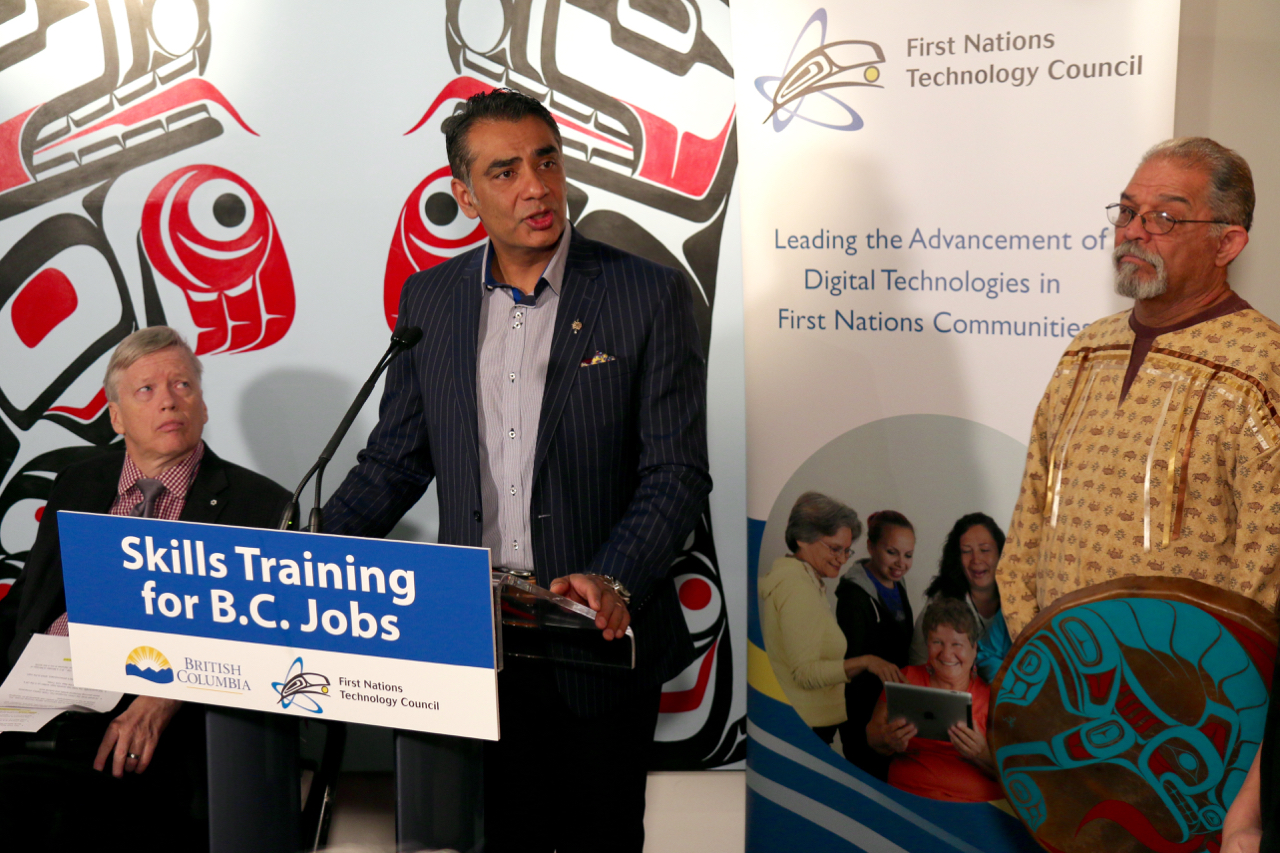The image depicts an indoor event centered around a presentation with three men prominently featured on a stage. The focal point is the man behind a lectern in the middle, speaking into a microphone. He has short black hair, light brown skin, and is dressed in a dark blue pinstriped suit adorned with a pocket square, over a light grey button-up shirt. His mouth is open mid-speech, and his hands rest on the lectern, which displays a banner reading, "Skills Training for Busy Jobs, British Columbia First Nations Technology Council."

To his left, another man with light skin and grey hair is seated, looking attentively up at the speaker. On the right side, there is an older man with white hair, a white mustache, and a beard. He is wearing traditional Native clothing and glasses, holding a round shield featuring a blue and red wolf design. He stands looking directly at the camera.

The backdrop includes a banner that reads, "First Nations Technology Council, leading the advancement of digital technologies in First Nations communities," accompanied by images of four women engaging with a tablet or laptop. The wall behind features Native styled drawings of various animals in red and black, partially obscured by the people on stage.